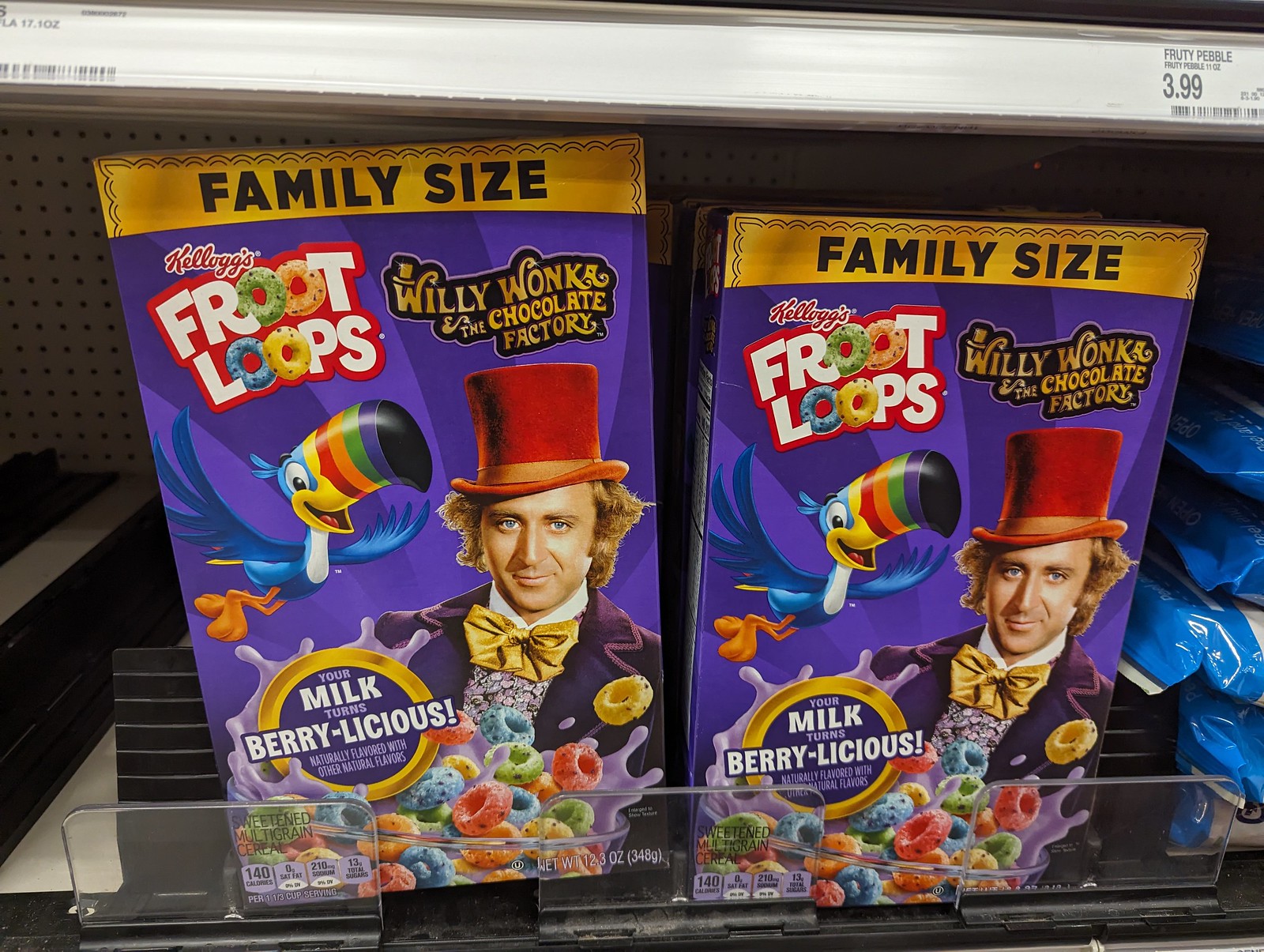The photograph captures a close-up view of a grocery store shelf, which is constructed from white metal and features a perforated back wall. Two large, prominently placed cereal boxes take center stage, flanked by a few blue plastic containers on the right side. The cereal boxes are Family Size Kellogg’s Froot Loops, distinguished by a yellow banner with black text at the top that reads "family size." Each box showcases a special edition design for Willy Wonka and the Chocolate Factory. On the left side of the box is the iconic Froot Loops toucan with its vibrant rainbow-colored beak. Beside the toucan is an image of the Willy Wonka character, adorned in a red top hat, purple jacket, and yellow bow tie, holding a bowl of colorful cereal with purple milk splashing out. Below this illustration, text announces, "your milk turns berry-licious, naturally flavored with other natural flavors." The vibrant cereal pieces in blue, orange, green, and yellow add a playful burst of color to the boxes, making them the focal point of the image.